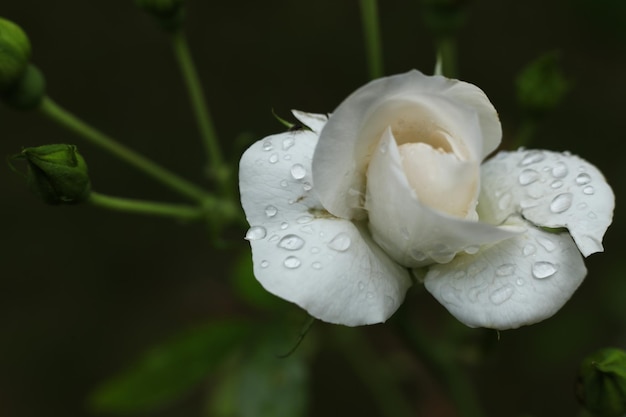This image captures a striking close-up of a white rose, prominently positioned to take up nearly half of the photograph. The rose, which hasn't fully bloomed, showcases delicate petals adorned with glistening dew or raindrops, suggesting an early morning or a recent shower. The central part of the flower, still slightly closed, reveals hints of yellow stamens peeking through. The background is mostly dark and out of focus, contributing to a stark contrast that elevates the rose as the focal point. Unopened buds and thick stems further populate the backdrop, alluding to the lush rose bush to which this singularly beautiful flower belongs. Notably, there are two unopened buds to the left and one additional bud at the bottom right. Large leaves can be discerned amidst the dark, abstract foliage, reinforcing the idea of a flourishing garden scene. The petals at the base of the flower stretch outwards, seemingly heavy with water droplets, emphasizing the lush and moist details of this captivating bloom.